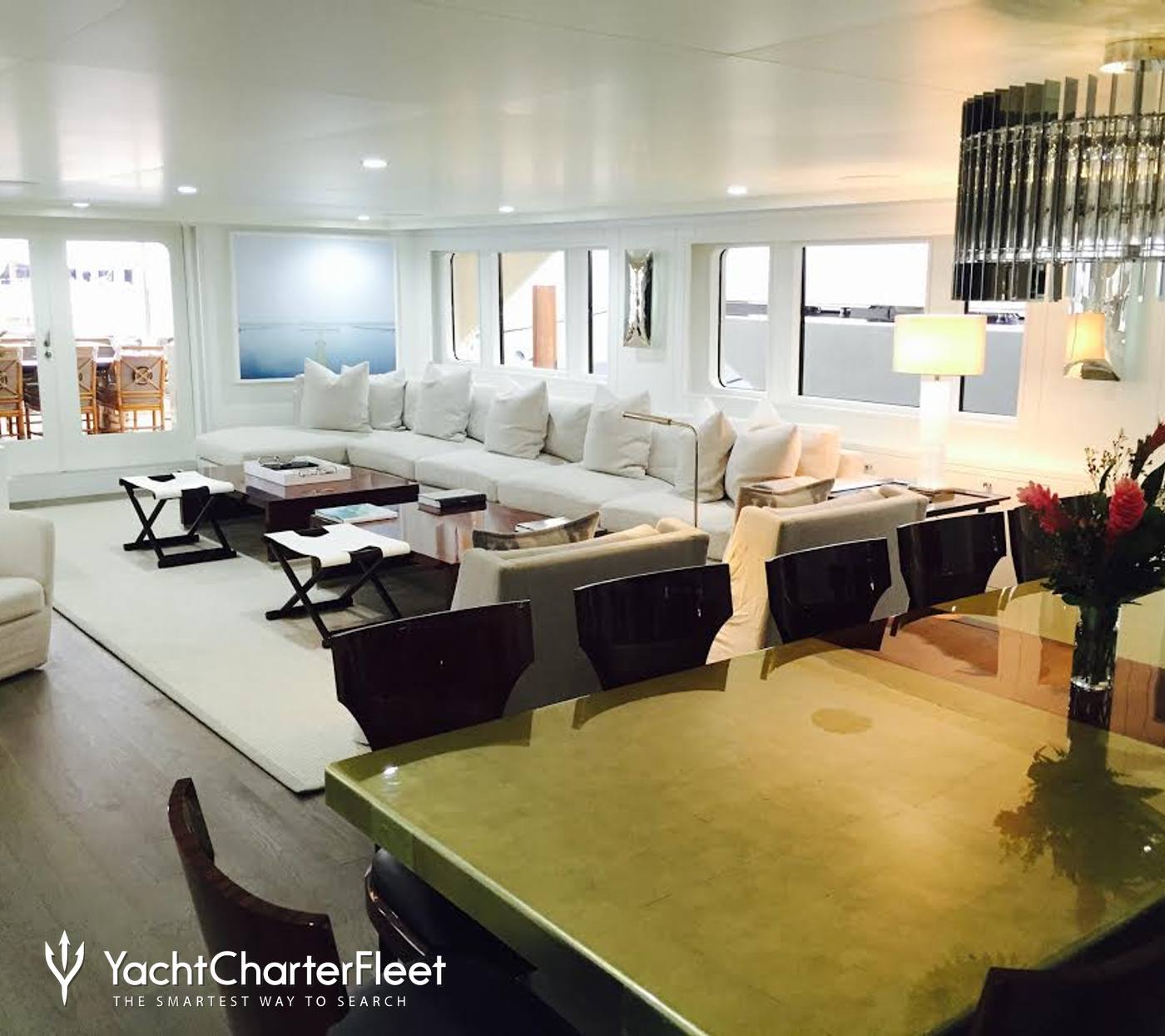This interior yacht advertisement showcases a luxurious and spacious setting with meticulous attention to detail. The room features white ceilings adorned with small white lights and is framed by expansive, white-trimmed glass doors on the far wall. To the right, a stunning large blue painting of the sea decorates the wall, leading to a corner with a modern silver chandelier illuminating a clear vase holding two vibrant pink roses, perched on a wooden table edged with green marble. In front of this table are five black high-back chairs, and to the side, a long plush white couch stretches across, accentuated with around ten white throw pillows. Nestled below the windows, which line the white wall, providing a view of water and distant buildings, is a sizable brown or wooden coffee table, laden with various books. A glossy dark wooden floor complements the setup, softened by a large, off-white throw rug situated in front of the couch. Completing the scene, the bottom left corner of the image features white lettering that reads "Yacht Charter Fleet," followed by the tagline "The Smartest Way to Search."